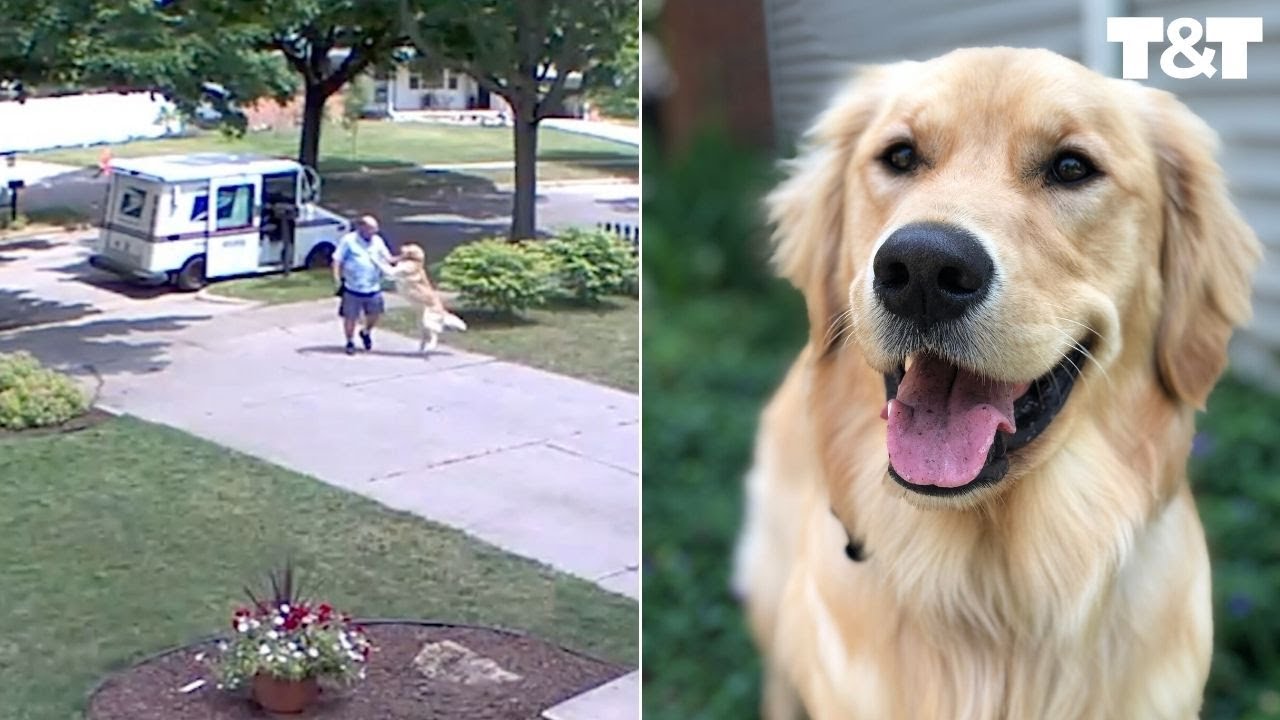This image is divided into two halves in a landscape orientation. The left side resembles home security camera footage, slightly blurry, capturing a friendly encounter in a driveway. A post office vehicle is parked at the end of the driveway, and a mailman, dressed in a light blue shirt and gray shorts, is walking up towards the home. He is warmly greeted by an excited, adult golden retriever jumping up to him with evident joy. The backdrop includes a neatly landscaped yard featuring two small shrubs flanking the driveway, a large tree, and a distinct half-circle flowerbed adorned with red lava rock, a sizable landscape boulder, and a terracotta pot overflowing with red and white petunias.

The right side of the image offers an intimate close-up of the golden retriever, capturing its expressive face and chest. The dog's mouth is slightly open, giving the impression of a happy smile. The background consists of soft, unfocused green shrubs, with a large white "T" and "T" logo in the upper right corner, adding a subtle graphical element to the scene.